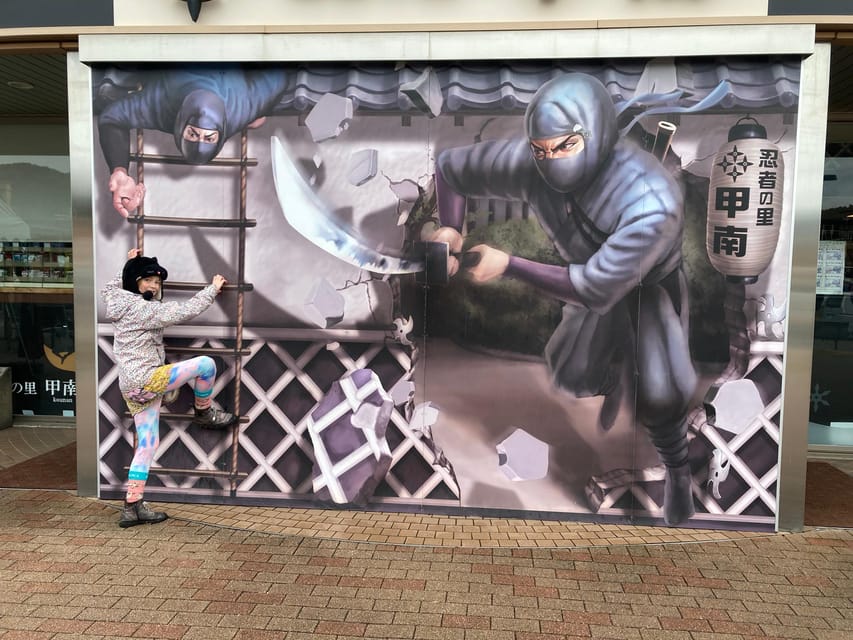This rectangular, landscape photograph captures a vibrant outdoor mural on a business's wall. Dominating the mural are two dynamic ninja figures: one descending from a rooftop in the upper left corner and another bursting through the wall to the right, wielding a large samurai sword. Both ninjas are dressed in classic attire, with their faces masked leaving only their eyes visible. The mural incorporates intricate details, such as a glimpse of greenery and a building behind the shattered wall, and a white thatch pattern at the base. 

To the right of the sword-wielding ninja is a white sign with Chinese lettering. The bottom third of the image shows a brick floor in tannish-red hues. Adding a playful twist to the scene, a young girl in colorful cloud-patterned leggings, an animal-style beanie, and a hoodie is posed on a real ladder that's leaned against the mural. She is climbing the ladder with one foot on the second rung and her hands gripping the sides, looking back at the camera with a bright smile, perfectly blending herself into the mural's action-packed narrative.